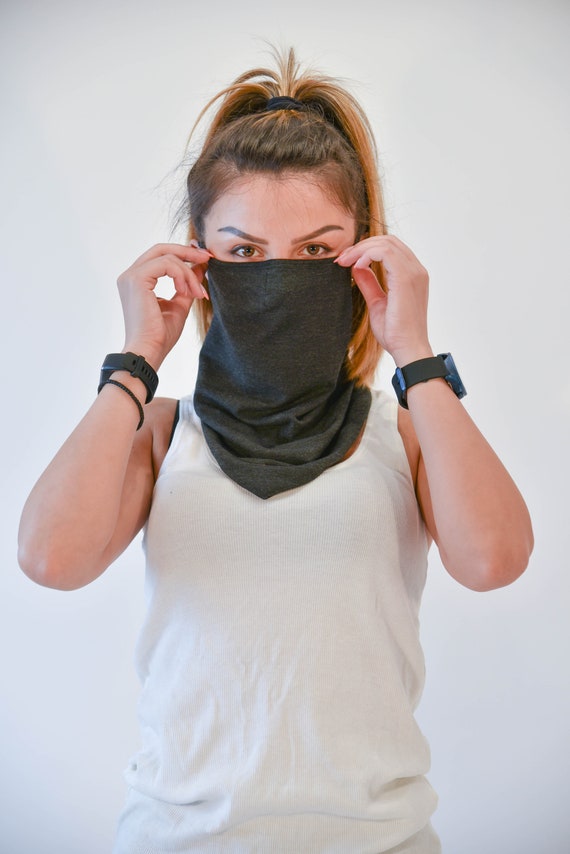The photograph captures a young Caucasian woman with light skin and brown eyes, looking directly at the camera. She has brown hair with orange highlights, pulled back into a loose ponytail. She is wearing a baggy white tank top and has a watch on each wrist. The focal point of the image is the woman adjusting a dark grey, gator-style mask over her face. She is pulling the mask up over her nose and mouth, with her fingertips grasping both ends of the fabric, positioned just beneath her eyes. Her expression is focused, and she appears to be mid-action, emphasizing both the functionality and possible stylistic intent of the face covering.